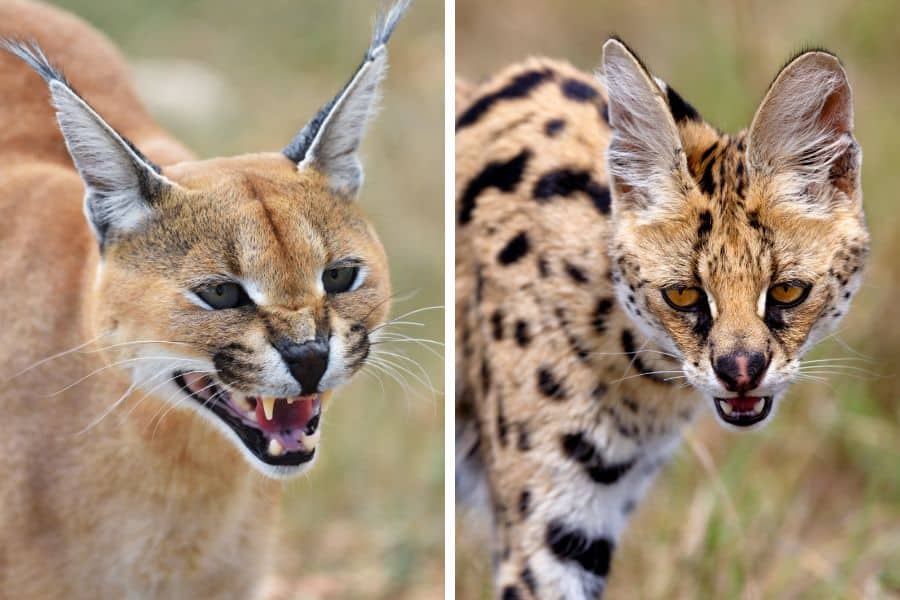The image features two side-by-side photographs of distinct wild cats set against blurred backgrounds featuring green and brown hues. In the left photograph, there's an animal resembling a Lynx with tufted, greenish ears, characterized by its open, snarling mouth which reveals sharp teeth and a red tongue. This cat-like creature has a predominantly brown body and dark eyes. In the right photograph, the animal displays a pattern similar to a hyena or a cheetah, with a brown body adorned with black spots and some white areas. This creature has large, rounded ears, orange eyes, and an open mouth that suggests it might be breathing rather than snarling, while it gazes slightly downward. Both animals are captured with high detail on their distinctive facial features and ears.